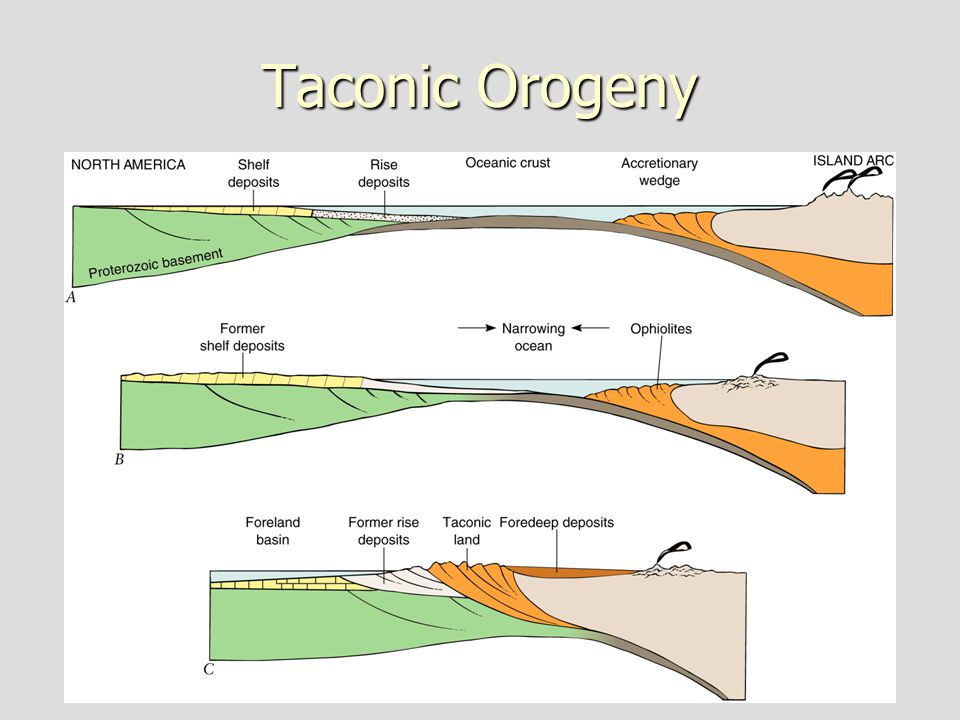The slide appears to be a visual representation from a PowerPoint presentation titled "Taconic Orogeny," displayed over a gray background. Its title is in light yellow letters at the top of the slide. Below the title are three sequential diagrams, each illustrating different stages of geographic and geological formations. 

At the top left of the first diagram, "North America" is indicated in black capital letters. This initial diagram, labeled as Figure A, features several color-coded sections including "Shelf Deposits" (yellow), "Proterozoic Basement" (green), "Rise Deposits" (white with black dots), "Oceanic Crust" (blue), "Accretionary Wedge" (orange), and "Island Arc" (brown). 

The middle diagram, labeled as Figure B, shows "Former Shelf Deposits" (yellow) and "Ophiolites" (orange), with "Narrowing Ocean" represented by two converging arrows. 

Finally, Figure C at the bottom, illustrates "Foreland Basin" (yellow), "Former Rise Deposits" (white), "Taconic Land" (orange), and newly formed deposits labeled as "Foredeep Deposits" (brown). This last diagram highlights a significant transformation where the ocean is no longer visible, and the formations are more compressed.

The colors used in the diagrams include green, yellow, blue, orange, and brown, providing a clear visual distinction between the different geological features and stages of the Taconic Orogeny.